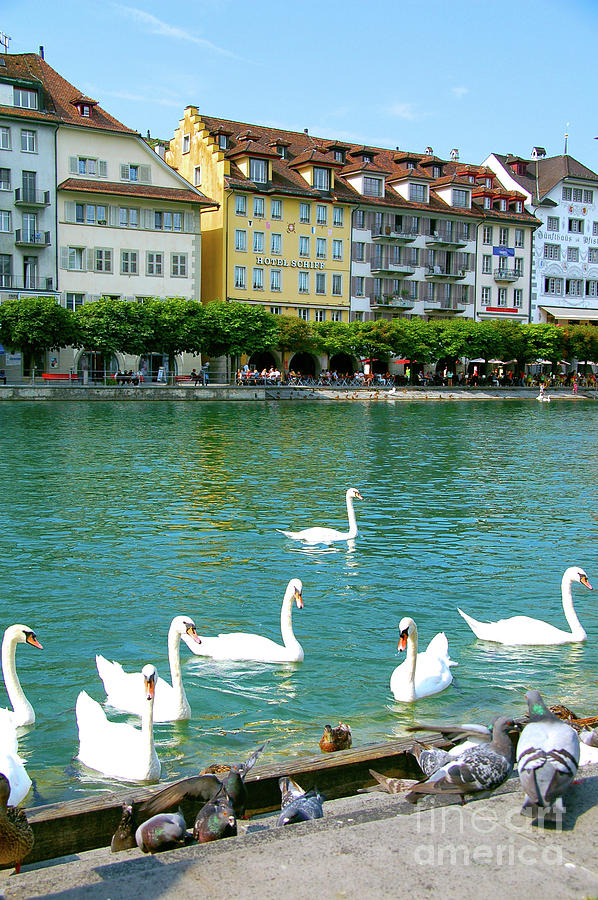This color photograph captures a picturesque European cityscape on a bright, sunny day. The scene features a tranquil marina lined with charming, multi-colored buildings, including a white, three-story building, a yellow hotel with "Hotel Shift" sign, and a beige building, each adorned with balconies. In front of these buildings, trees form a neat line, adding a touch of greenery. The marina's calm waters are home to a variety of birds—seven graceful swans gliding across the surface, alongside a brown duck and some white geese. Pigeons and doves congregate on the concrete steps leading down to the water in the foreground. People can be seen enjoying the serene atmosphere, sitting at tables with umbrellas near the water's edge. The scene is framed by blue skies overhead and the text "Line Art America" is subtly inscribed at the bottom of the image.